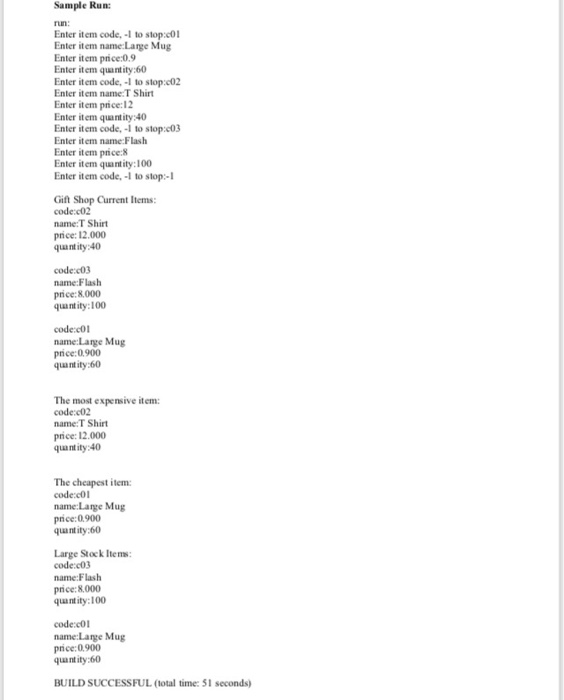The image features a white background with black text, resembling a coding output related to a website development project. At the top, there is a sample run section that lists item code information and item name details. Below this, there is a segment titled "Gift Shop Current Items" which further details codes, item names, prices, and quantities of various products. 

Following the item listings, the image identifies the most expensive item in the inventory: a T-shirt priced at $12. The cheapest item is then highlighted as a large mug, priced at $9. Additional stock items are cataloged beneath these sections. 

The image concludes with a statement indicating that the build was successful, with the total time taken being 51 seconds. Overall, this image encapsulates information pertinent to the coding and construction of a website’s inventory display, providing a snapshot of item details and system performance metrics.